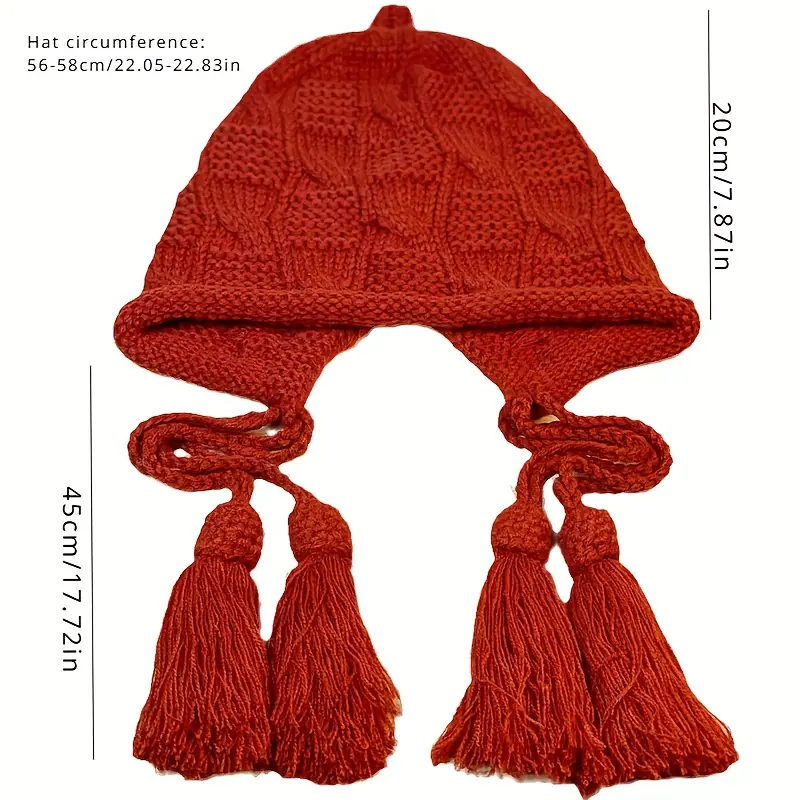The image showcases a handmade, dark orange (or red) knitted cap on a white background. The cap features two triangular ear flaps, each with large, stringy tassels hanging down the sides. There are also two braids with tassels extending from the ear flaps. The hat’s measurements and dimensions, written in black text, provide detailed sizing information: a circumference ranging from 56 to 58 centimeters (22.05 to 22.83 inches), a height of 20 centimeters (7.87 inches) noted in the top right corner, and a vertical black line on the bottom left side indicating 45 centimeters (17.72 inches). This meticulous description ensures accurate understanding of the cap's size and appearance.